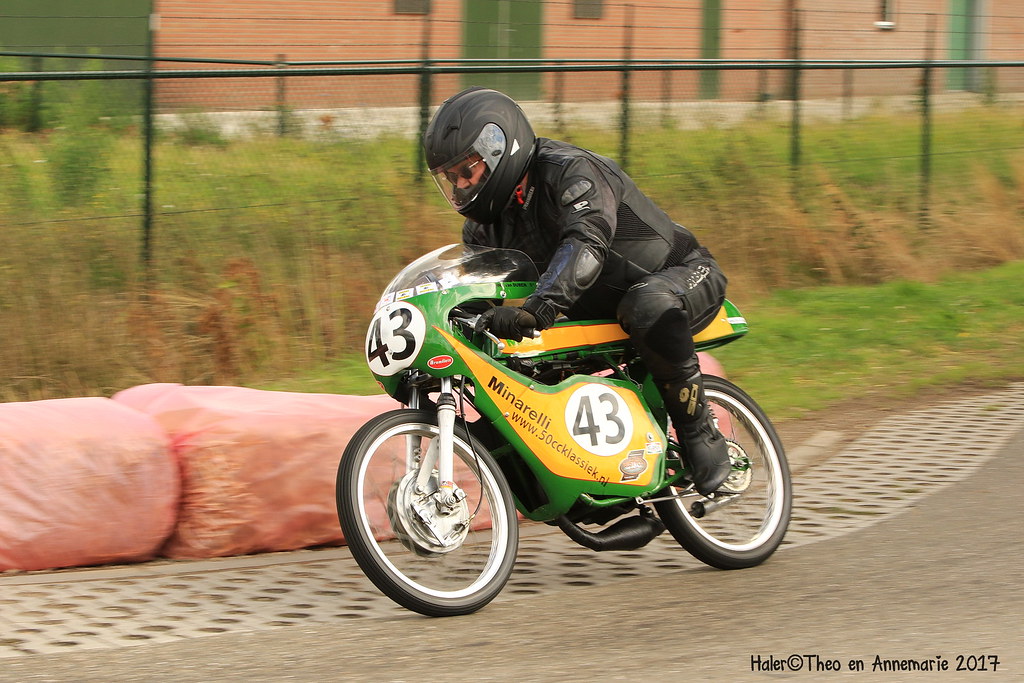The image depicts a male rider on a green and yellow Minarelli racing motorcycle, marked with the number 43 in bold black letters on a white circle, visible on the side and front of the bike. The rider is fully equipped with a black helmet, black gloves, black full-body racing leathers, black boots, and a low visor that just covers his eyes, over which he wears sunglasses. He is leaning into a curve, possibly on a dirt track, with evidence of crash protectors like pink stuffed bags behind him. A reinforced fence with black posts and tall grass appears in the background, with a long brick building with green doors stretching across the top of the image. The lower right-hand corner of the photograph is marked with the text "Holder Thiel and Anna Marie 2017." The entire photograph, a commercial image measuring about eight by six inches, emphasizes the dynamic motion and safety preparations of the racing scene.